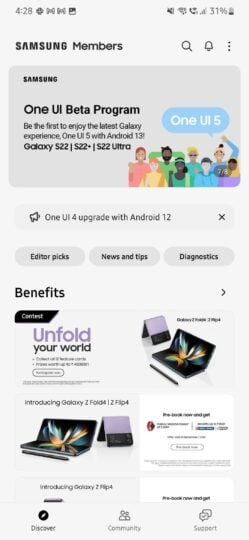Screenshot of the Samsung Members App on a Mobile Device

The image is a screenshot from a Samsung mobile device displaying the interface of the Samsung Members app. At the top of the screen, the app's title "Samsung Members" is prominently displayed. Below this title, there is a section providing general information about the benefits offered by the Samsung Members program. 

The screenshot further includes a subheading titled "Benefits," which likely expands on the perks available to members. Additionally, there is another subheading titled "One UI Beta Program." This section invites members to join the One UI Beta Program, allowing them to be among the first to experience One UI 5 with Android 13. 

However, the text displayed on the screenshot is partially cut off or obscured, making it difficult to read all the details and fully understand the specific offerings and benefits of the Samsung Members program from this image alone.